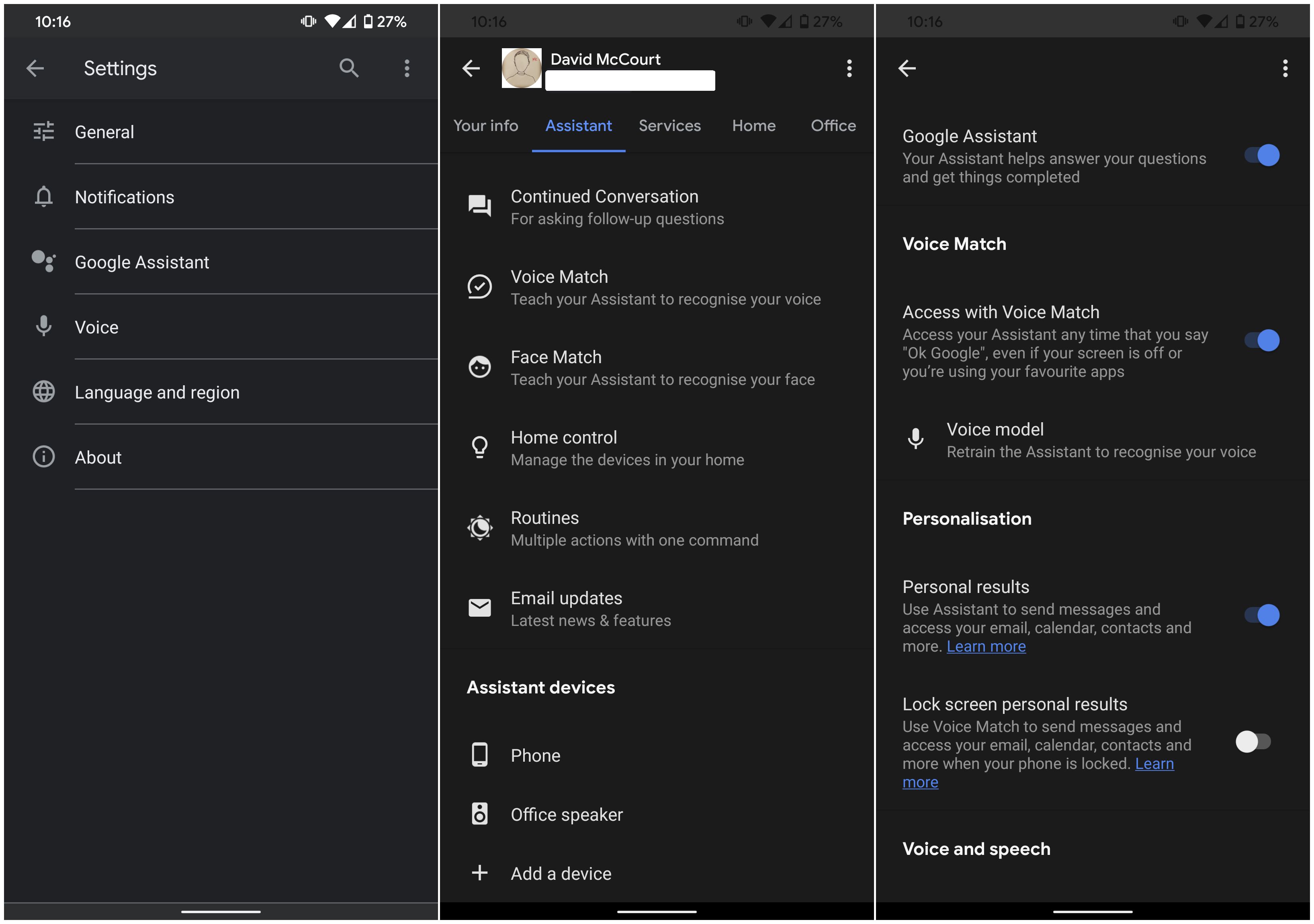This image is a screenshot collage of three smartphone screens, each depicted in dark mode with black backgrounds. The system clock on all three screens shows a time of 10:16 AM, and the battery level stands at 27%.

The first screenshot on the left displays the device's Settings menu. The user has accessed a drop-down list featuring various settings options. From top to bottom, the list includes: "General," "Notifications," "Google Assistant," "Voice," "Language and Region," and "About."

The middle screenshot highlights a profile page for a user named David McCourt, suggesting that this is the smartphone's owner. This screen is focused on the "Assistant" tab of the profile settings, displaying numerous customization options such as: "Continue Conversation," "Voice Match," "Face Match," "Home Control," "Routines," and "Email Updates." The "Assistant Devices" section lists connected devices including "Phone," "Office Speaker," and an "Added Device."

The third screenshot on the right pertains to Google Assistant's Voice Match settings, which allow access and personalization via voice recognition. Indicated options include setting up and managing voice commands and interactions through the assistant.